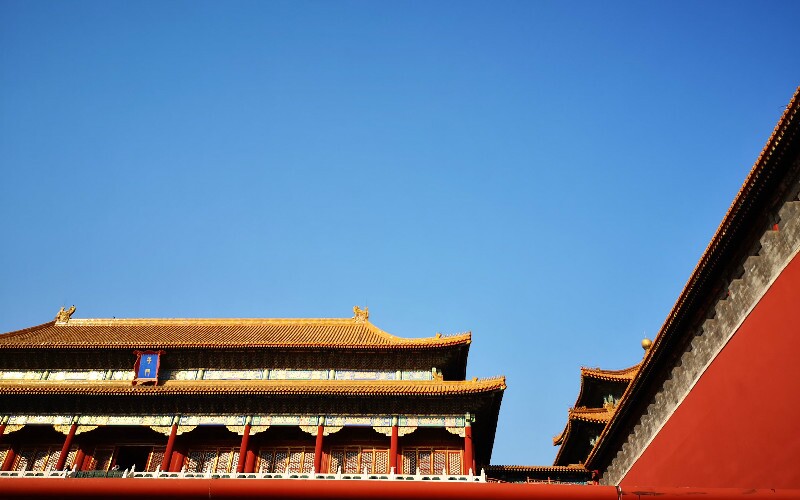The image is a detailed photograph of an ancient temple or traditional Asian building, likely of Japanese or Chinese architectural style. The structure stands majestic with its vibrant red walls and brown roofing. The photo is taken from the ground level looking up, capturing the multiple-tiered levels adorned with intricate decorations. The roof is a striking golden-yellow, possibly made of clay tiles, and is decorated with statues that resemble mythical animals. Red columns extend from one floor to the next, adding to the temple's grandeur. Ornate symbols, possibly Mandarin or Japanese, embellish the building, enhancing its cultural significance. The scene is set against a bright, clear blue sky without any visible people or additional imagery, emphasizing the serene and timeless beauty of the temple. White railings accentuate the lower levels, providing a stark contrast to the rich colors of the structure.